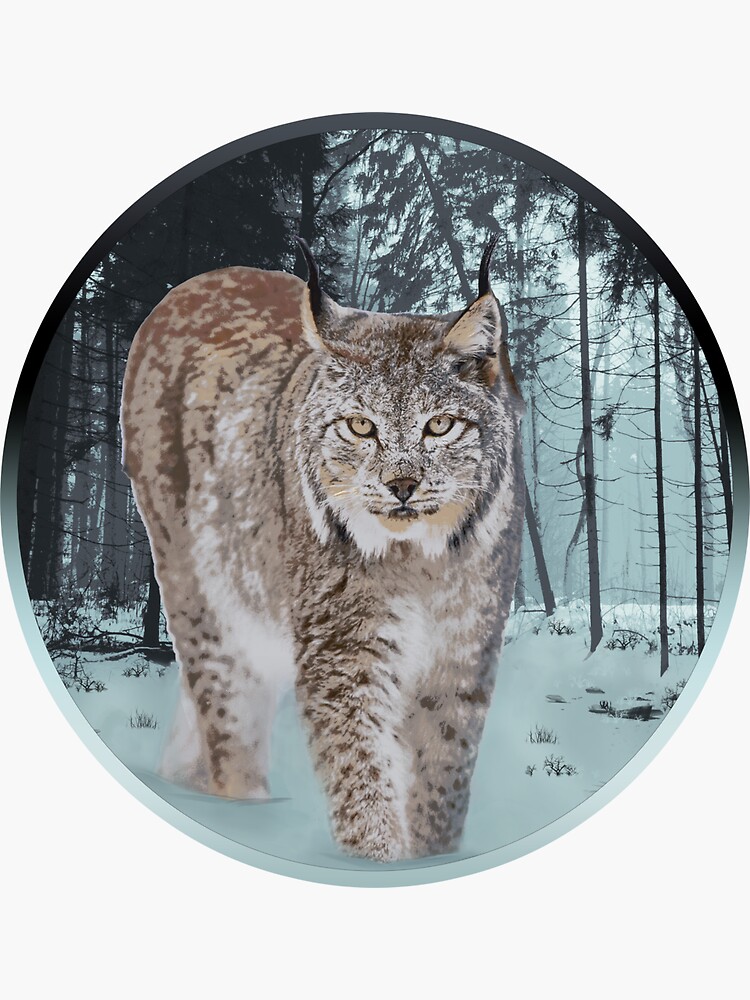This detailed photograph is encased within a circular frame on a white background, capturing a mesmerizing winter scene in a snowy forest. At its center, a majestic lynx stands in the snow, facing directly toward the camera with light greenish-yellow eyes that pierce through the foggy surroundings. The lynx's fur exhibits a beautiful blend of gray and brown, adorned with darker speckles, and a white belly and inner legs. Its distinctive cat-like face features upright ears tipped with characteristic tufts of extended hair. The backdrop of the image reveals an ethereal, fog-laden forest dotted with spruce trees, enhancing the wild and serene atmosphere of the scene. This image vividly portrays the lynx's powerful presence and the tranquil, yet slightly mysterious, ambiance of its natural habitat.